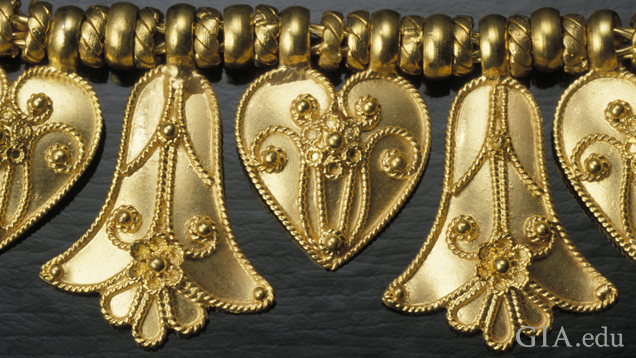This close-up image showcases an intricate piece of jewelry, potentially a bracelet, composed of a thin gold chain adorned with a series of gold rings and ornate pendants. The chain displays a repeated pattern of smooth, solid gold rings alternating with rings etched with diagonal, rope-like patterns. 

Suspended from the gold rings are five visible pendants: three heart-shaped and two bell-shaped designs. The hearts, positioned at the leftmost, middle, and rightmost points, feature elaborate gold braiding on their edges, extending inward to form swirl patterns that culminate in petite flower motifs. The bell-shaped pendants, situated between the hearts, are equally detailed, with flower designs and teardrop shapes that resemble blossoms fanning out.

The image is taken against a backdrop of black, leather-like material with a slight sheen, adding contrast to highlight the jewelry’s golden hues. In the bottom right corner, the watermark "GIA.EDU" is inscribed in light gray letters, indicating the source of the image. The leftmost and rightmost hearts are partially cut off, emphasizing the close-up nature of the photograph and focusing attention on the detailed craftsmanship of the jewelry.